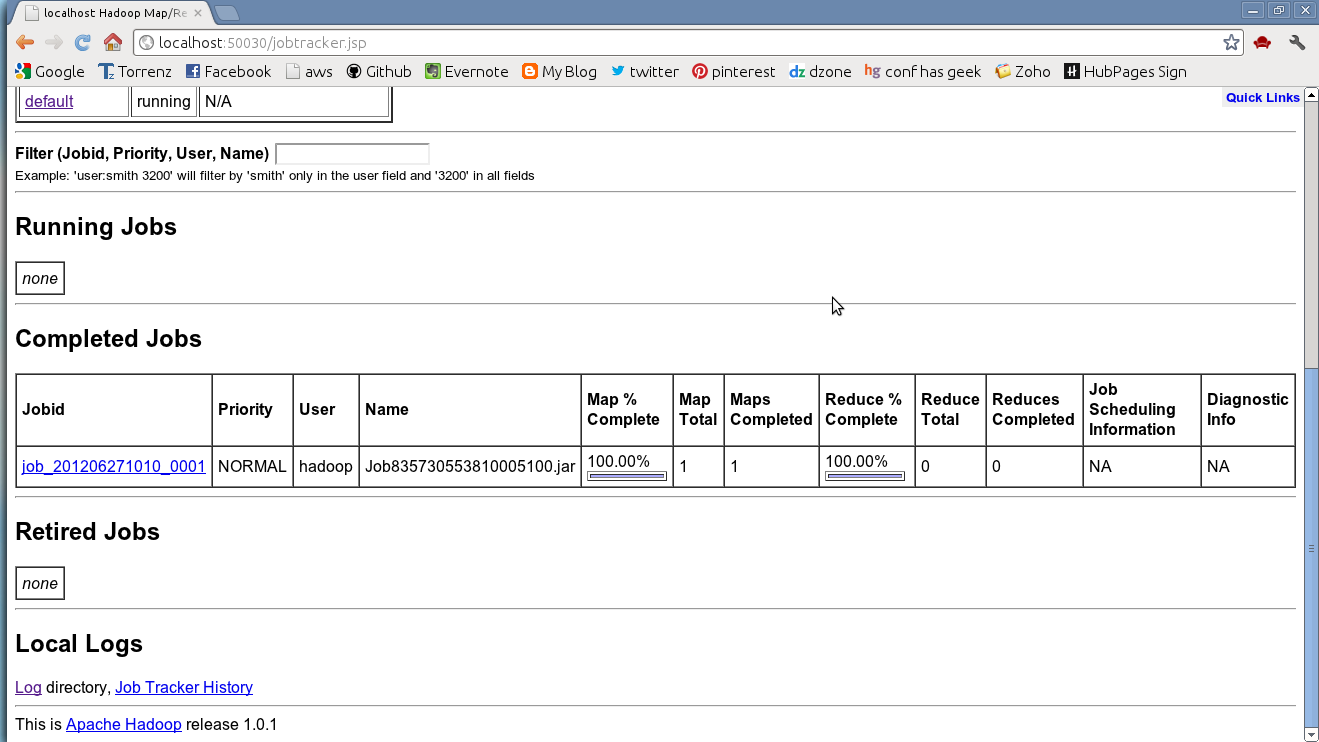This image is a screenshot of a computer screen showcasing a software interface, likely related to job or task management. It features a user-friendly and organized layout with several distinct sections:

- The top portion of the screen is a blue-gray horizontal rectangle, which appears to be the browser window's frame. On the left side of this frame is a tab with black text, indicating the current active window.

- Directly below the tab is a navigation toolbar containing several icons: an orange left-pointing arrow, a grayed-out right-pointing arrow, a blue reload circle, followed by a large search bar.

- Underneath the toolbar is a list of favorite links or bookmarks.

- The main content area of the screenshot starts with what looks like an invoicing section. In the upper left corner, bolded black text reads "Filter," followed by details in parentheses: "job ID, priority, user name." Next to this, there is a data entry box.

- Below the "Filter" box, there's a small-printed example.

- Further down, there is another section header in bolded text saying "Running Jobs." About two lines below this heading, there's a white square bordered in black with the word "None" written inside it.

- A gray horizontal line divides the "Running Jobs" section from the "Completed Jobs" section.

- The "Completed Jobs" section contains a grid-like structure. The grid headers, all in bolded black text, include: "Job, Bid, Priority, User Name, Map % Complete, Map Total, Maps Completed, Reduce % Complete, Reduce Total, Reduce Completed, Job Scheduling Information, Diagnostic Info." Below this header, there is only one line of job-related information displayed.

- On the lower left of this grid, another bolded black heading "Retired Jobs" is displayed, followed by a white square with the word "None."

- The bottom section of the screenshot features a "Local Logs" header in bolded black text.

This detailed layout effectively organizes various job statuses and diagnostic information for easy accessibility and readability.